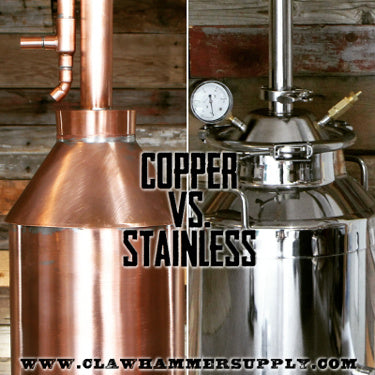The image is a comparative guide featuring two side-by-side photographs showcasing different types of distilleries. In the center of the image, bold black text with white borders reads "copper versus stainless," highlighting the primary focus of the comparison. Both distilleries are set against a backdrop of light brown wooden planks.

On the left side, the copper distillery stands out with its warm, bronze hue and shiny reflective surface. The copper still features a round canister base that tapers upward, transitioning into a large copper pipe extending vertically from the top.

On the right side, the stainless steel distillery is characterized by a sleek, gray-silver finish. It boasts additional features such as side handles, numerous clasps, and a circular pressure gauge with a black dial and white notches. The canister is cylindrical, similar to the copper version, but includes more practical accessories for ease of use.

Both stills are designed for alcohol production, such as brewing or fermenting beer. At the bottom of the image, the website "www.clawhammersupply.com" is displayed in black text with white borders, running from the left to the right corner, indicating the source of the comparison.